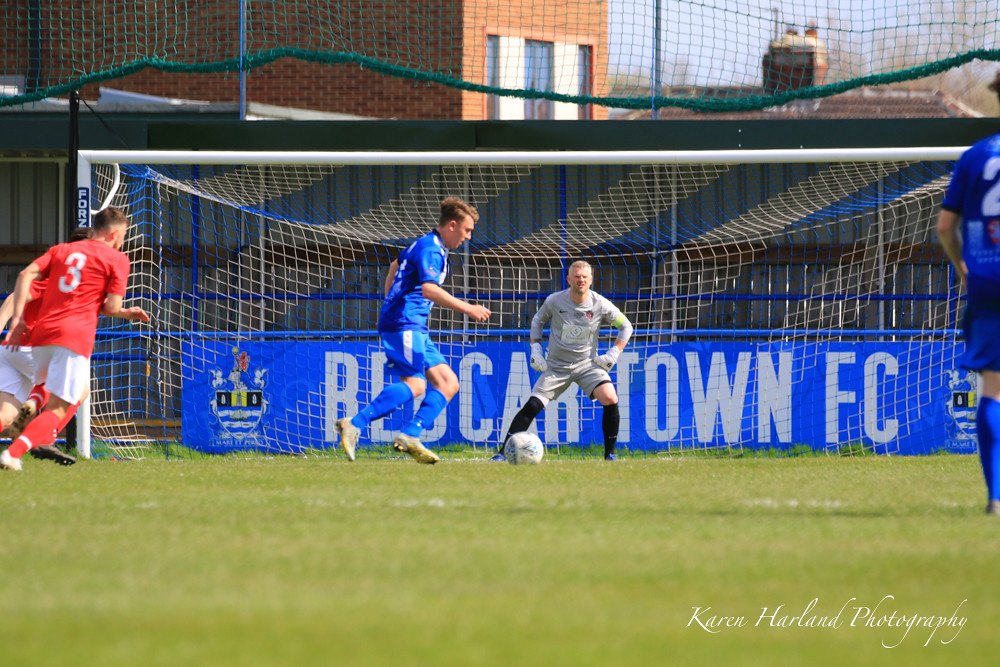In this vibrant, full-color outdoor photograph captured by Karen Harland Photography, a lively soccer game unfolds on a sunlit day. Set against a backdrop of clear blue sky, a chimney, and a combination of red and brown brick buildings, the scene is anchored by a large soccer net in the center. The net is being defended by a player in a white uniform, while a blue-clad player is poised to kick the ball towards the goal. To the right, another blue player, whose number remains partly obscured, looks on. The field, lush with green grass that stretches up towards the middle of the image, is flanked by a royal blue banner in front of the net, indicating the football club, although the text is partially hidden by the players. Additionally, a red player, wearing number three, is captured running towards the action, with his back facing the camera. The photograph, rectangular in shape and taken from a level viewpoint on the field, includes a watermark at the lower left corner that reads "Karen Harland Photography."